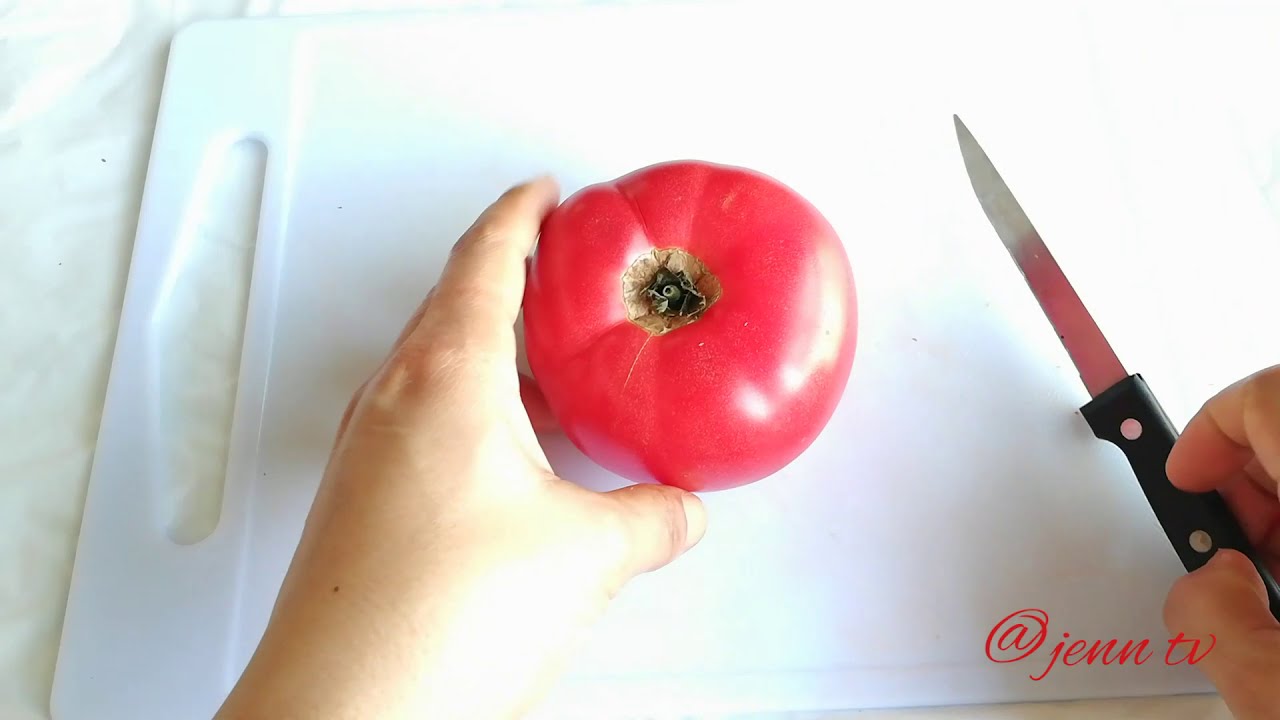The image captures a detailed scene of a culinary preparation, featuring hands cutting a tomato. A pale-skinned person is holding a bright, reflective red tomato on a white plastic cutting board with their left hand. They are using a small, sharp paring knife with a black handle in their right hand, poised to cut the tomato. The cutting board is situated on a white, granite-like countertop with a light, marble texture. The tomato's stem has been removed, but a stubby brown leaf remains visible where the stem used to be. The light source shines from the top, highlighting the tomato and casting a shadow on the hand to the lower right. In the bottom right corner, the red cursive text '@GenTV' is visible, possibly indicating the source of the image. This scene likely originates from or is a still from a cooking video.